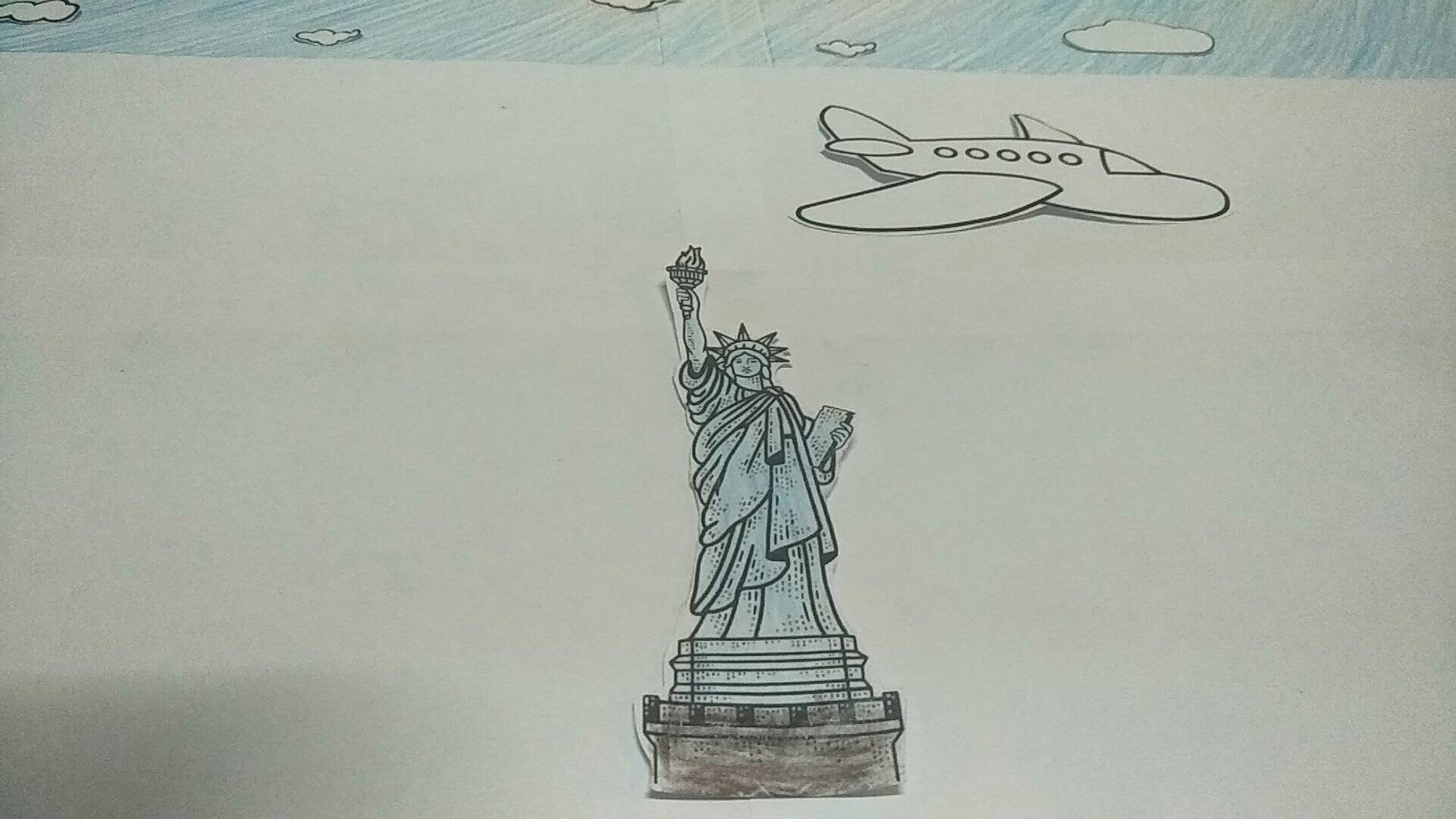A meticulously detailed line drawing of the iconic Statue of Liberty is presented, showcasing the statue standing majestically on its pedestal. The background is a minimalistic grey, allowing the artwork to stand out prominently. The statue itself, including Lady Liberty's flowing robes and serene facial features, is rendered in striking black ink with a delicate pale blue tint, adding a subtle hue to her distinguished appearance. The pedestal is depicted in brown, with intricate details including five or six raised sections resembling a balustrade, enhancing the architectural authenticity.

Above the statue, a plane is illustrated soaring through the sky. The aircraft, drawn in black ink, features numerous cabin windows, contributing to the realism of the scene. Fluffy white clouds, meticulously shaded against the light blue sky, add depth and dimension to the celestial backdrop. The overall composition combines elements of meticulous line work and selective coloring, creating a harmonious and visually engaging piece that pays tribute to one of the world’s most recognizable monuments.